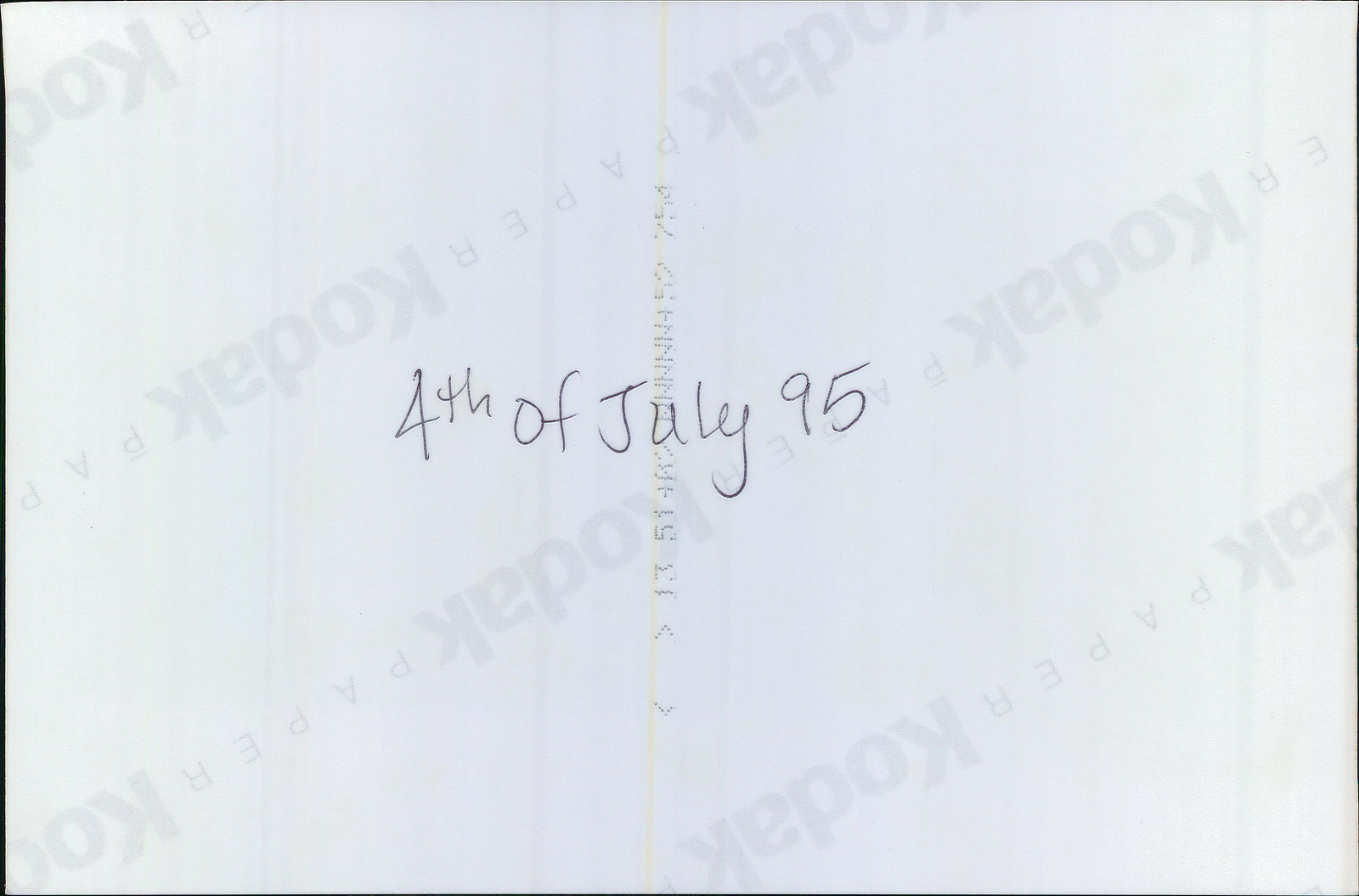The image features a small photograph, approximately 4x6 inches in size, which has been flipped over to reveal its back side. The back of the photograph is marked with diagonal strips showcasing the words "Kodak paper" printed repeatedly, indicating the brand of the photographic paper. This Kodak paper label appears upside down. In the center of the back side, a black ballpoint pen inscription is visible, reading "4th of July, 1995." Additionally, there are alphanumeric codes printed across the photograph by the printer, signifying various technical details such as color and density settings. The photograph was processed with normal settings, implying that the negative was developed without any color corrections or adjustments.